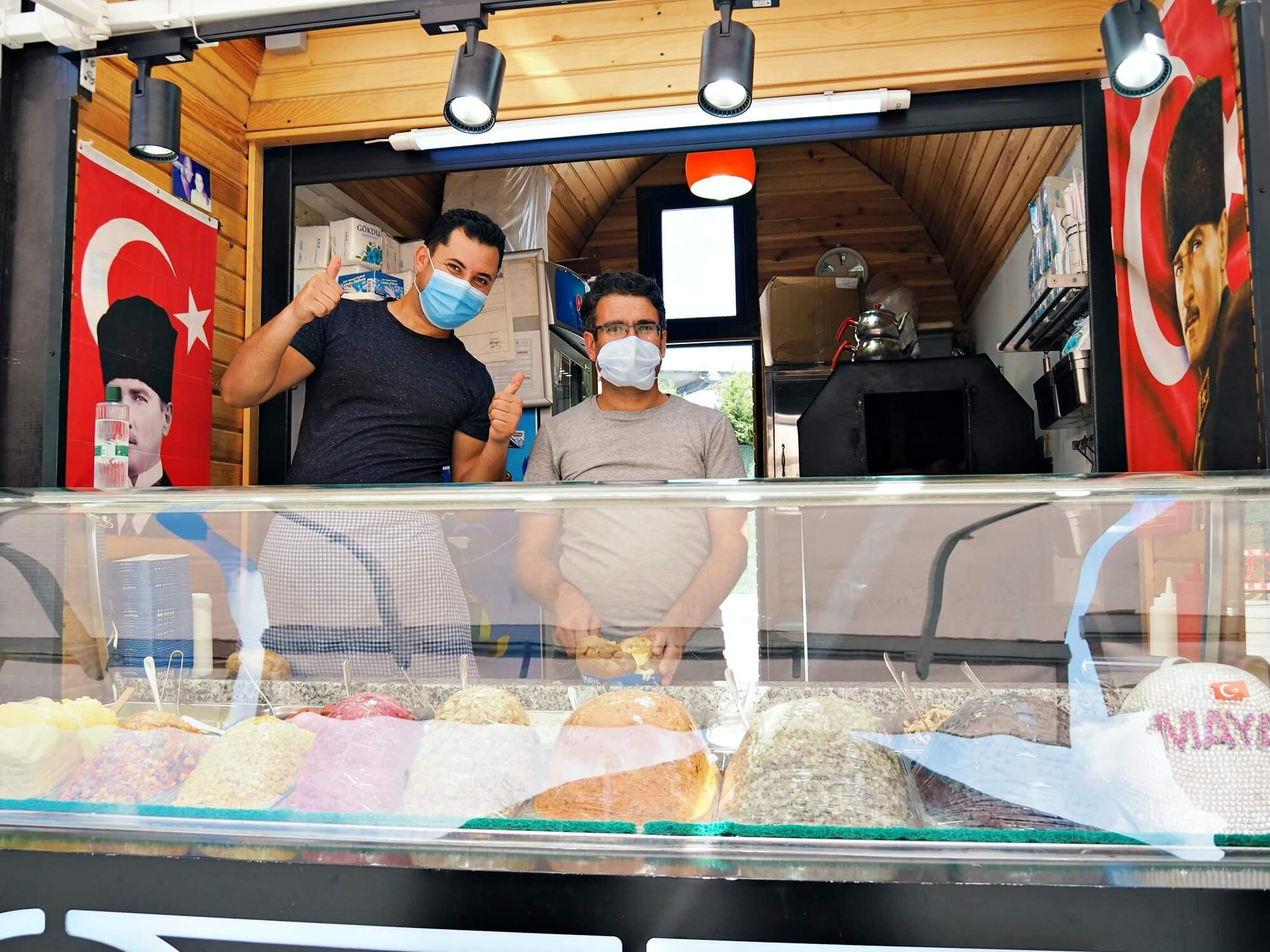In the image, there's a vibrant food truck with a clear glass countertop displaying various food items, potentially meats, for sale. The truck's interior is made of wood and is decorated with Russian posters featuring a red background, a crescent moon, and a star, and possibly portraits of significant figures like leaders or actors. Two young men, likely the owners, are standing behind the counter. The individual on the left, dressed in a black t-shirt, is giving a thumbs-up signal, his blue mask highlighting a twinkle in his eyes. The other, slightly shorter, wears a gray t-shirt, a white mask, and glasses, appearing to prepare food. Both men, appearing cheerful, are facing the customers. On either side of them are Coca-Cola machines, and the work area behind them is stocked with silver pots, shelves filled with supplies, and necessary appliances for their business. Additionally, there's a mark or sign in the right-hand corner with the letters "M-A-Y," possibly indicating a brand or label. The food truck provides a colorful, inviting atmosphere for passersby to view and purchase food directly from the display.